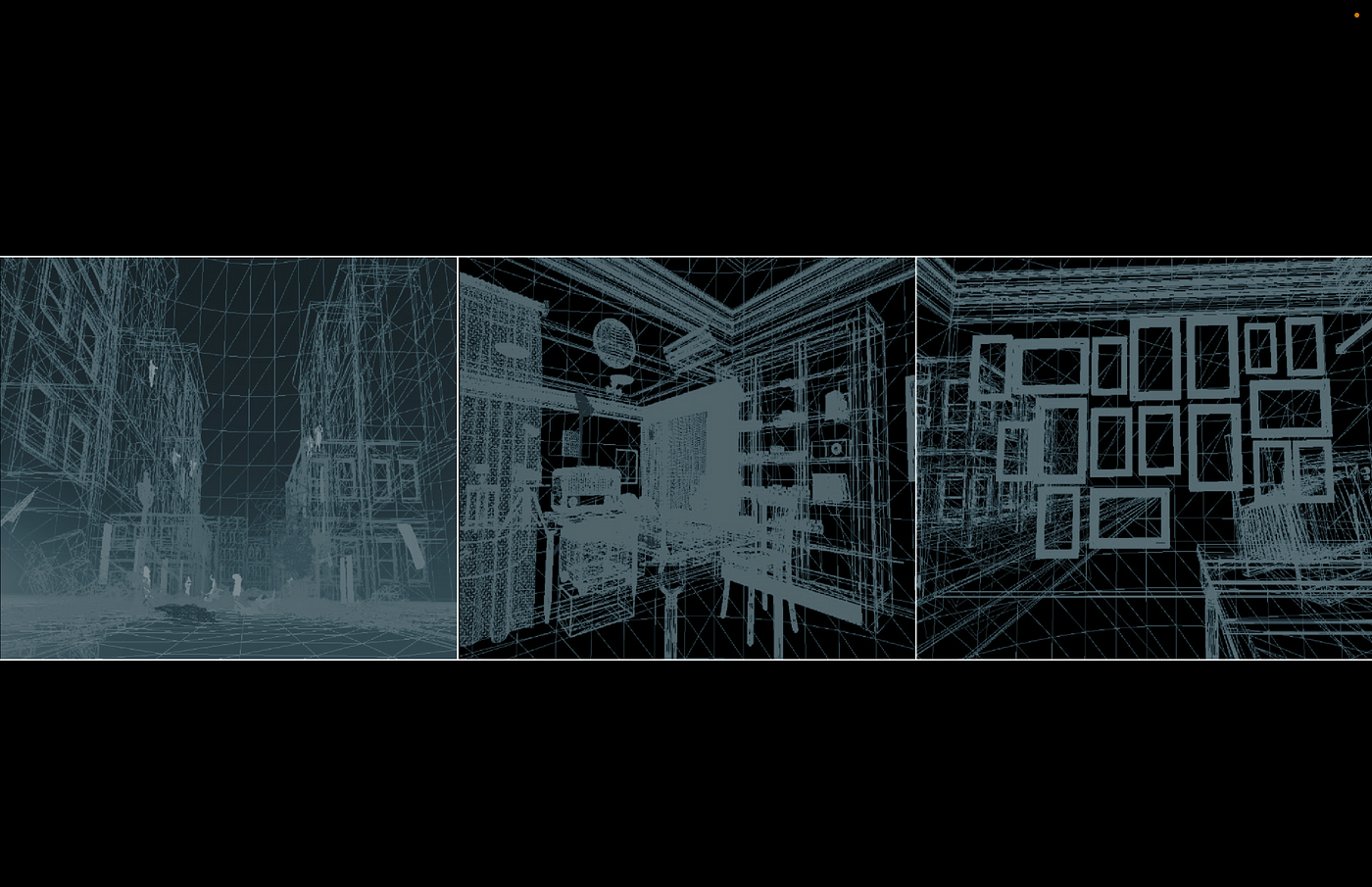The image features a triptych of computer-generated environments, each rendered in intricate black and teal line work, reminiscent of x-ray or mesh visualizations. The left-hand section depicts an outdoor city scene with buildings lining both sides of the street, populated by indistinct figures. The middle image portrays an interior space, likely an office or kitchen, with a desk, a clock on the wall, a shelf, and a cabinet. Details such as a curtain, possibly next to a stove, and a chair in front of the shelf add depth to the scene. The rightmost picture shows a wall adorned with numerous empty picture frames and a table with an indeterminate object on it; the wall appears transparent, allowing glimpses of the exterior buildings. The overall effect is a set of environments defined by minimalistic, yet detailed, white lines against a stark black background, creating an impression of seeing through walls.